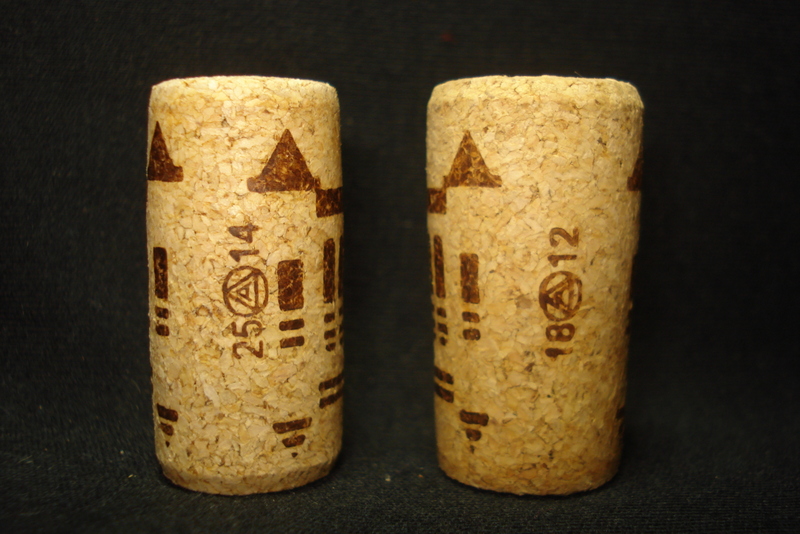This color photograph, taken in landscape mode with a very close-up and slightly magnified perspective, focuses on two cork wine stoppers resting on a black, soft-textured background resembling carpeting or felt. The image captures the corks at eye level, showcasing their tan, beige color characteristic of traditional cork material, accentuated with darker brown markings. Both corks feature similar designs with variations in their number codes and symbols. The cork on the left displays the numbers "25" and "14," with a circle containing the letter "A" imprinted between the numbers. The right cork bears the numbers "18" and "12," also featuring a circular stamp with the letter "A" in the middle. Both corks are decorated with an array of geometric patterns including triangles, horizontal lines forming triangular shapes, and elongated rectangles. The black background includes a few specks of dirt, emphasizing the detailed texture captured in the photograph.